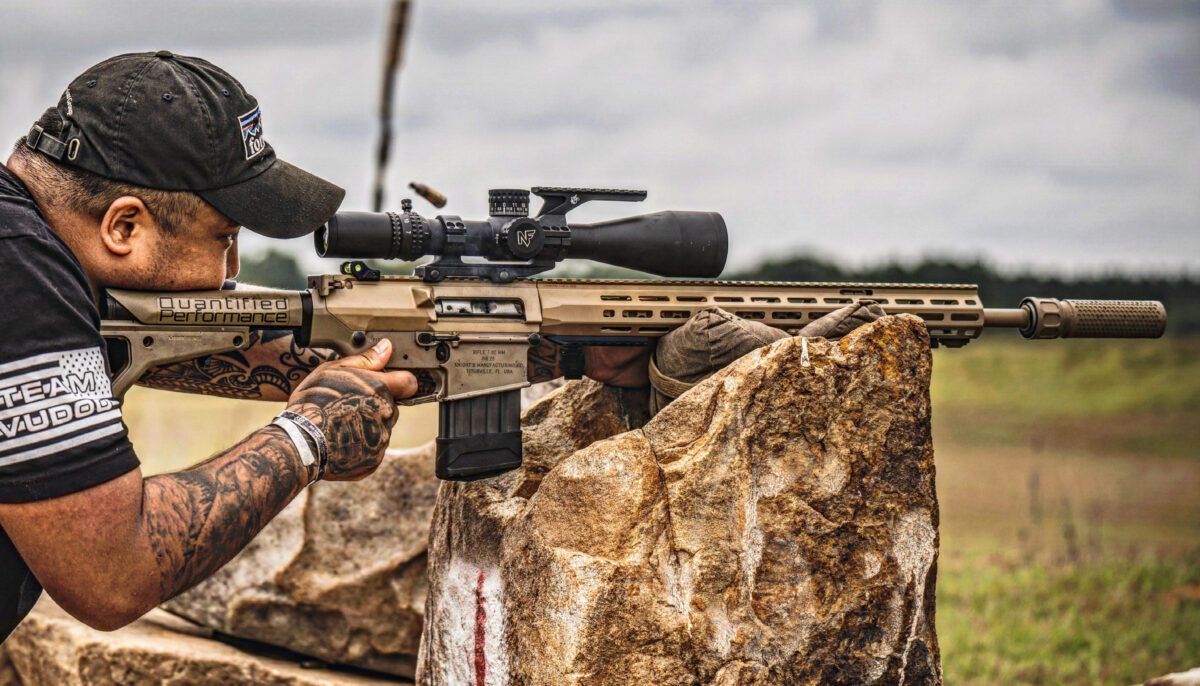The image captures an outdoor scene featuring a man engaged in target practice with a high-caliber rifle. The sky is overcast with gray tones and scattered white clouds, suggesting a cloudy day. The man, dressed in a black t-shirt and a matching black ball cap with an adjustable back, has tattoos covering both his forearms. His shirt bears the inscription "Team Vudoo" alongside a black and white American flag on the right sleeve. 

The rifle he holds is substantial and long, possibly a .50 caliber, equipped with a prominent black scope and a silencer. Its body is a light brown to metallic shade and features ridges on the muzzle, indicative of gas release functionalities. The black magazine clip and stock butt are also visibly part of the rifle’s design. The man has the rifle steadied on a large, brown-gray rock, supplemented by some bags for additional support. 

As he peers through the scope to aim, a brass shell casing is seen ejecting from the other end of the rifle, indicating he has just fired a shot. The foreground includes green grass and a brown dirt road, while a blurred tree line forms the backdrop. This detailed setting highlights the intense focus of the man and the precision of the equipment in an outdoor shooting environment.